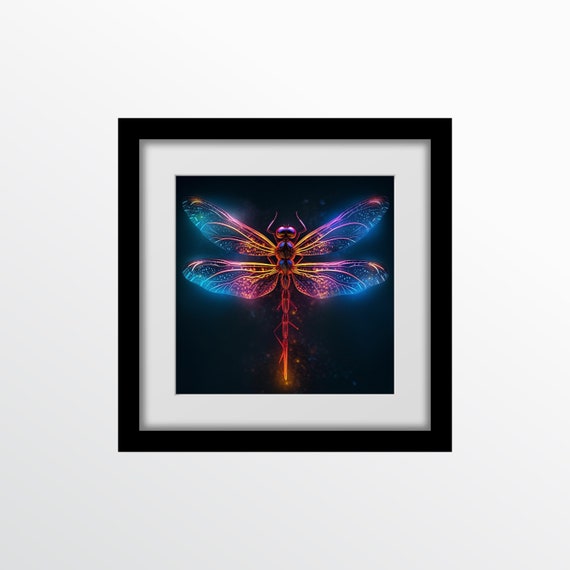The image portrays a vibrant piece of artwork displayed in an art museum, showcasing a dragonfly rendered in striking neon colors. The dragonfly is centrally positioned within a black square frame, which is further accentuated by a white mat. Set against a black backdrop, the dragonfly features intricate details: its body transitions from a neon red to an orange hue towards the tail, and it has antennae that extend towards the top of the picture. The wings are a spectacular blend of neon blue, pink, and orange, with the upper wings pointing towards the upper corners and the lower wings spreading out towards the middle of each side. The background of the entire frame is white, enhancing the vividness of the dragonfly's colors. The overall effect is a visually striking and detailed portrayal of a dragonfly in a display that catches the eye with its luminescent quality and meticulous presentation.